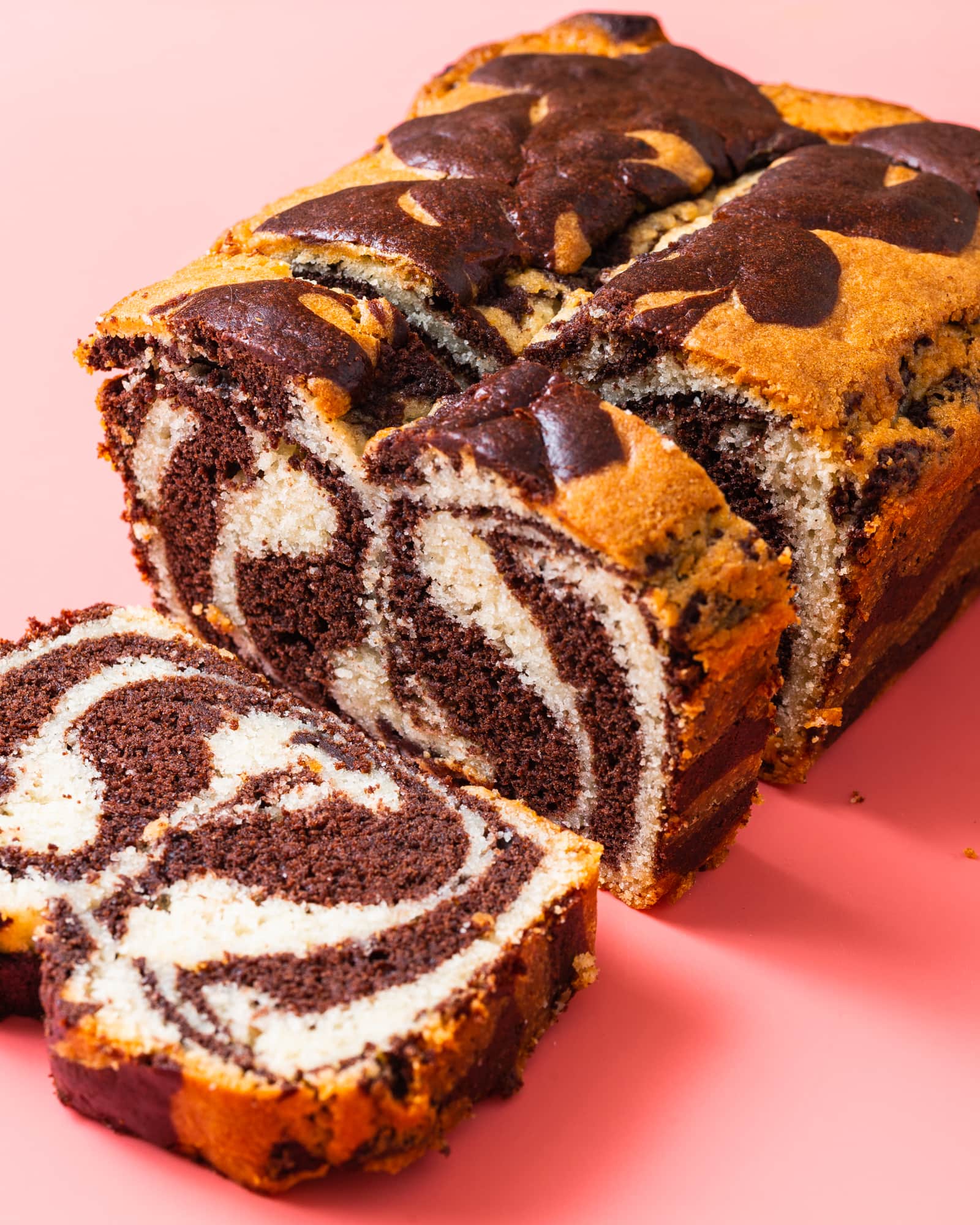This image showcases a close-up of a delicious-looking marbled bread that appears akin to a cake roll or Bundt cake. The loaf, prominently displayed, is cut into multiple pieces, with one piece lying flat on a white table and another piece standing upright. The rest of the bread remains uncut. The exterior of the bread is beautifully browned with intricate chocolate swirls. Inside, the bread reveals a striking, even swirl pattern of white and black, hinting at a chocolate and vanilla mix. The top of the bread features a dark chocolatey pattern, possibly with a hint of orange glaze, giving it a vibrant, glossy finish. The bread seems to emit a reddish glow on one side due to the lighting, and shadows cast by the cut pieces lend a dark pink hue to the scene. Scattered crumbs on the table add a touch of rustic charm to the image.